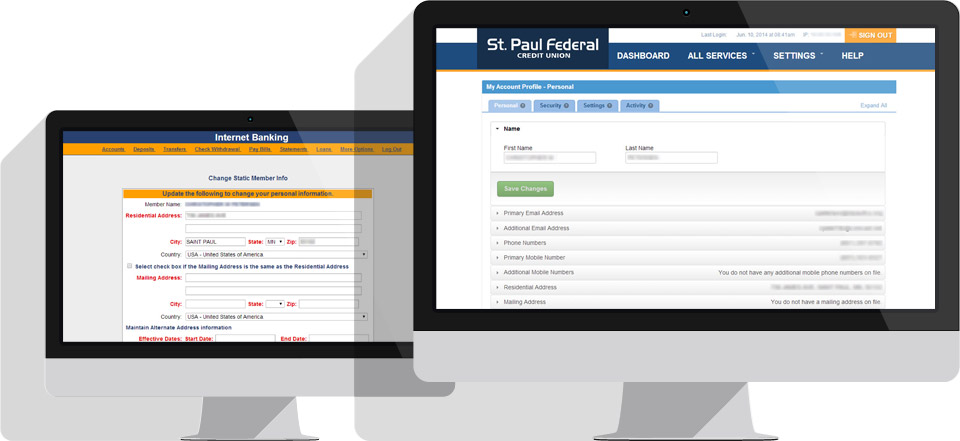On the left side of the image, a computer monitor displays the dashboard of the St. Paul Federal Credit Union's online banking system. The dashboard provides various options for internet banking, including accounts overview, deposit and transfer services, check withdrawals, bill payments, and statement reviews. The interface appears to allow users to change static member files, update their information, and modify personal details such as permanent residential address, city, state, zip code, and country. This process includes filling out fields and checking site boxes, with a manager sending confirmation emails to update the user's residential and mailing addresses.

The top left section prominently shows the organization's name, "St. Paul Federal Credit Union," along with a summary of all available services, settings, and health status. It also indicates the user's last login date as June 12, 2014. An orange button labeled "Sign Up" seems to be available for new account creation.

The dashboard offers features related to personal security, settings, and tracking recent activity. It has fields for the user's first and last name, position, primary email address, and phone numbers. Notably, it specifies the primary phone number and highlights that there are no additional mobile phone numbers on file. 

The interface seems organized into several rows and columns, although the details in some of the rows on the right are blurry and hard to read. The monitor itself has black bezels and is set against a lower part that is silver with a subtle shadowing effect.